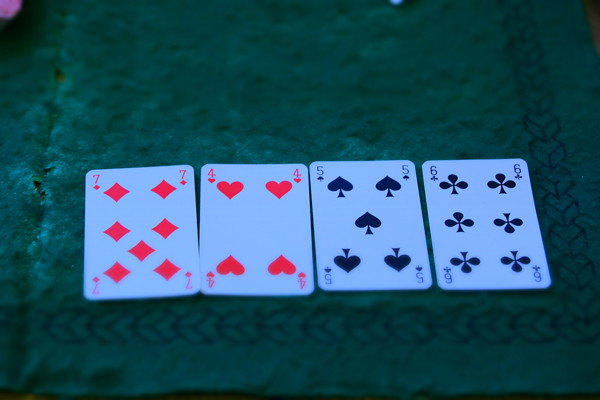A detailed photograph captures four playing cards laid face-up on the plush, green velvet surface of a card table. The photograph is taken from a corner angle, revealing an ornate black pattern that adorns the right and bottom edges of the table. The cards, arranged side-by-side, showcase a seven of diamonds with its vivid red diamond symbols prominently displayed. Next to it is the four of hearts, featuring four red heart symbols. The third card in line is the five of spades, marked by five bold, black spade symbols, followed by the six of clubs, which shows six black club symbols. Notably, the lower quarter of the image appears slightly blurry, possibly due to a filter effect, causing the numbers and symbols at the bottom of the cards to look out of focus. This slight distortion draws attention to the texture and detail of the card table surface, emphasizing the rich, velvety fabric.